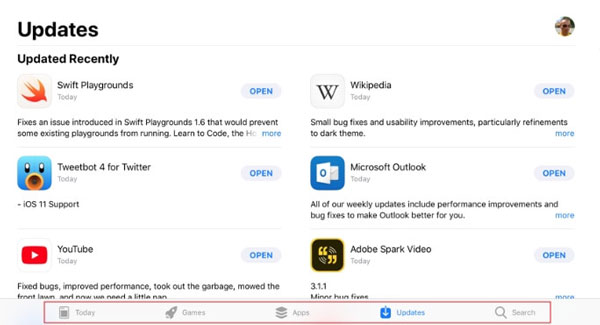The image showcases a notification screen highlighting recent updates for various apps. In the top left corner, bold black text reads "Updates." To the right of this text is a very small, barely distinguishable circular profile picture of a person wearing sunglasses. Under the "Updates" heading, smaller text notes, "Updated Recently."

The list of updated apps is as follows:

1. **Swift Playgrounds:** 
   - **Text:** "Today"
   - **Button:** "Open"
   - **Description:** Fixes an issue introduced in Swift Playgrounds 1.6 that would prevent some existing playgrounds from running. Learn to code.

2. **Tweetbot for Twitter:** 
   - **Icon:** Image of a bird with its mouth open
   - **Description:** iOS 11 support.

3. **YouTube:** 
   - **Button Icon:** Red box with an arrow pointing right

4. **Wikipedia:**
   - **Icon:** Letter "W" inside a box

5. **Microsoft Outlook:** 
   - **Icon:** A white box inside of a blue square
   - **Description:** All of our weekly updates include performance improvements and bug fixes to make Outlook better for you.

6. **Adobe Spark Video 3.1.1:**
   - **Icon:** A black box with yellow colors inside

This detailed notification screen provides a clear overview of recent app updates and their key features or fixes.